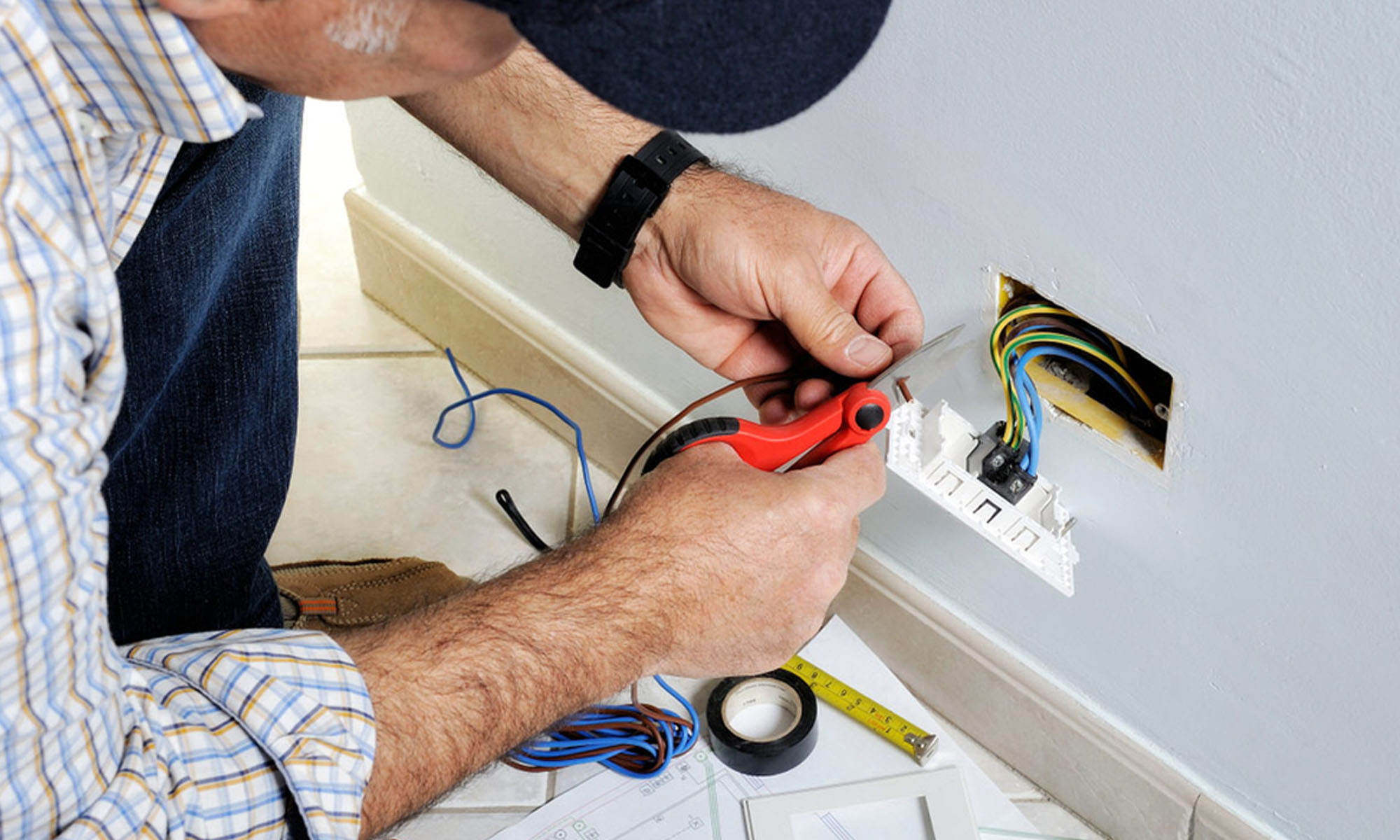The image depicts an older man, identified by his white facial hair, meticulously working on an electrical fixture. He is using a pair of scissors with red handles to cut a brown wire emerging from a white contraption hanging off a gray-blue wall. This contraption, resembling an electrical outlet, is crowded with around ten different colored wires, suggesting a complex setup. The man, only partially visible, is wearing a plaid shirt with blue, white, and some orange stripes, rolled up sleeves, blue jeans, and a black watch on his left wrist. He appears to be bent down, possibly kneeling, with one of his brown shoes and a bit of his leg visible. Additional items such as a tape measure, black electrical tape, and extra wires lie on the white tile floor around him, indicating a detailed and organized electrical repair or installation task. A leather tool belt is partially seen below his right hand, further emphasizing his readiness for the task at hand. The overall scene suggests a focused moment in a domestic or office repair setting.